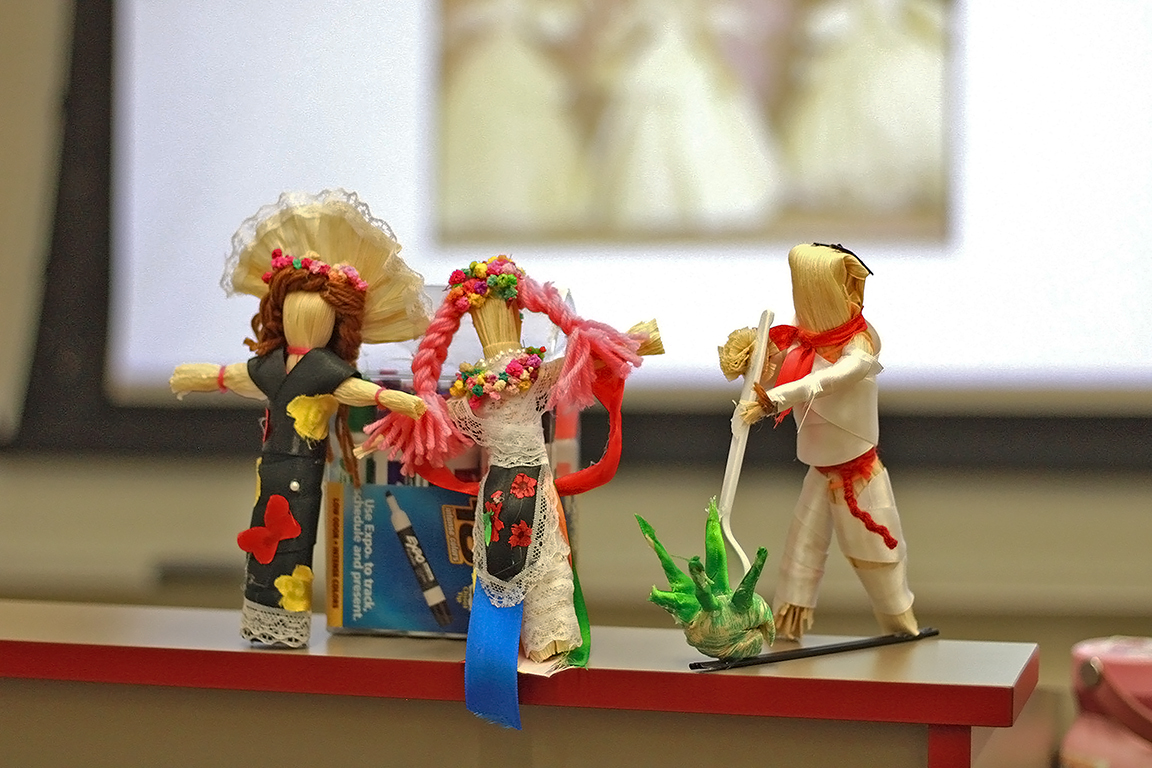In the image, three handmade fabric doll figures, resembling faceless voodoo dolls, are intricately arranged on a reddish-brown ledge. The surface of the ledge itself is light brown with dark red edges. Each figure stands out distinctly:

1. The first figure on the left features brown hair and is adorned in a black dress decorated with red butterflies, with the bottom portion of the dress being white. It appears to be made from straw and fabric.

2. The middle figure showcases pink hair tied in knots and wears a lacy white dress. It is accessorized with flowers in its hair and a black, white, and red flower strip that has blue elements.

3. The final figure on the right is dressed in an all-white outfit with a red belt or scarf. This figure has a bag over its head and holds a white, straw-like pipe leading to a green head with protruding green horns below it.

In the blurred background, a large, indistinct white screen is visible, and next to the figures, there is a pack of Expo Magic Eraser markers. The dolls stand out sharply against the blurred backdrop, highlighting their detailed, fabric-constructed designs.